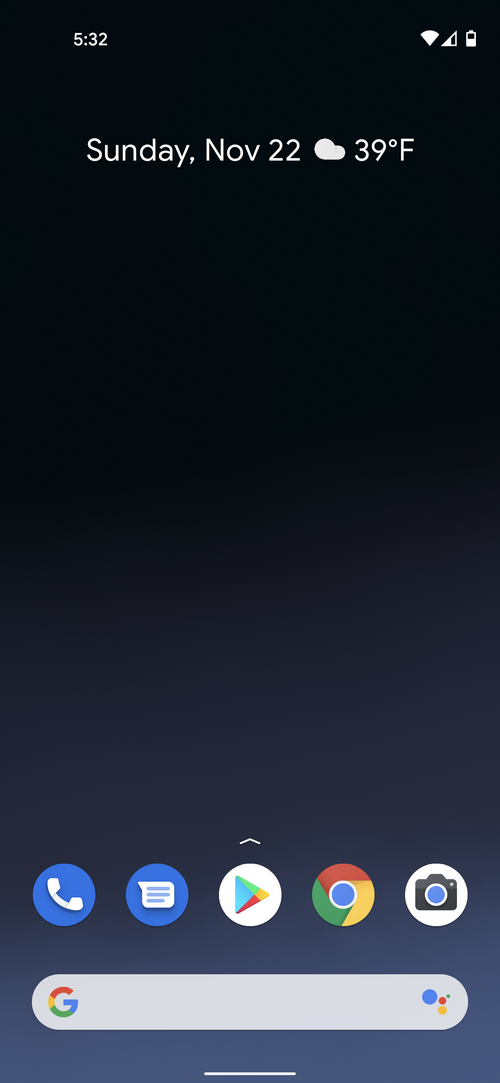The screenshot showcases a smartphone home screen with a gradient background that transitions from black at the top, through lighter gray in the middle, to a medium gray with a bluish tint at the bottom. In the top left corner, the time is displayed as "5:32." On the top right corner, there are icons for Wi-Fi connectivity and battery status. Below these icons, the date "Sunday NOV 22" appears in white text, accompanied by a cloud icon and the temperature "39°F," indicating that it's a cloudy day on Sunday, November 22nd.

At the bottom of the screen, there are five app icons neatly arranged. From left to right, these include: a phone icon in white and blue, a messaging icon in blue with a white speech bubble, the Google Play icon with a multicolored arrow, the Google Chrome icon featuring a circle with red, green, yellow, and blue colors, and a camera icon on a white background. Below these icons, the Google search bar stretches across the screen with the recognizable "G" logo on the left and four small dots on the right. At the very bottom, there is a short horizontal light gray line, likely indicating a touch gesture area for accessing additional features or navigation.